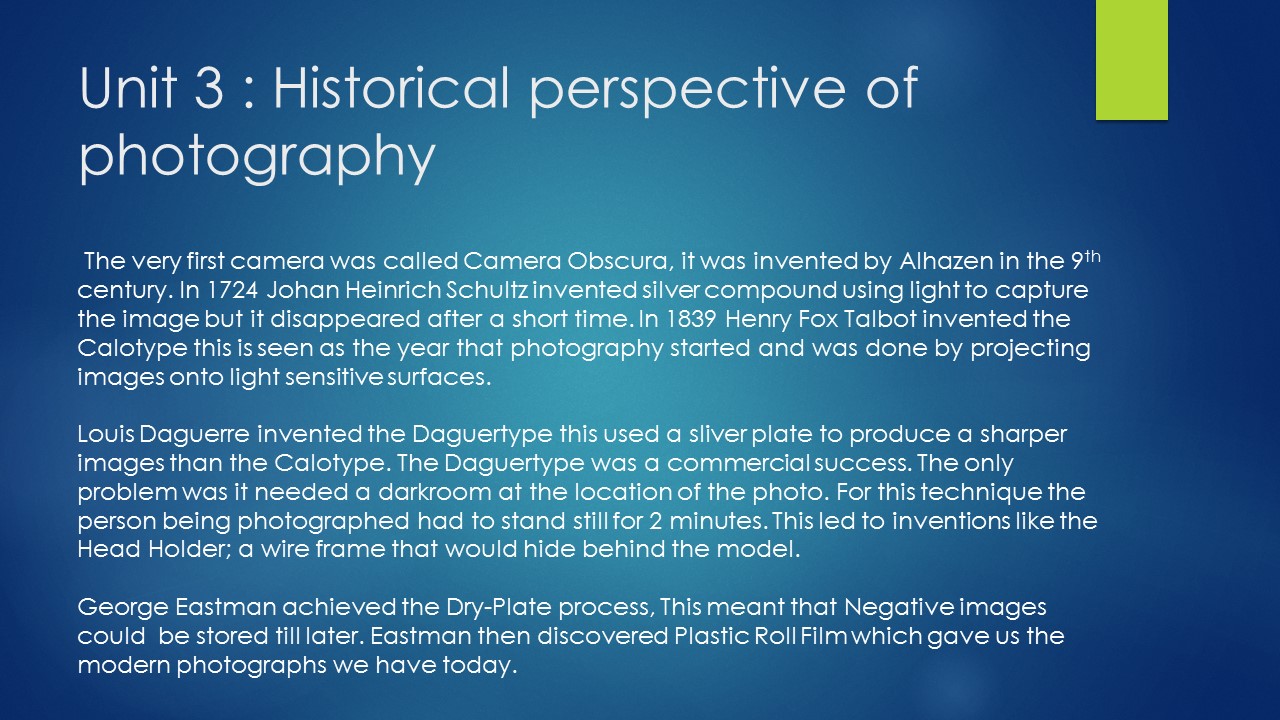The image displayed in the slide is from a PowerPoint presentation with a blue background and white text, entitled "Unit 3, Historical Perspective of Photography." The slide, which is formatted in the shape of a high-definition television (wider than it is tall), features a small olive green vertical stripe near the upper right-hand corner, descending to about the level of the word "photography."

The text is well-spaced across the slide and includes several paragraphs that chronicle key milestones in the history of photography. It starts with the invention of the Camera Obscura by Alhazen in the 9th century. It then mentions Johann Heinrich Schultz, who in 1724 developed the silver compound technique to capture images which would disappear quickly. The timeline continues to 1839 with Henry Fox Talbot’s invention of the Calotype, marking the beginning of modern photography by projecting images onto light-sensitive surfaces.

Further advancements are noted, such as Louis Daguerre’s invention of the Daguerreotype, known for its sharp images produced on a silver plate, but requiring a darkroom and long exposure times. George Eastman’s development of the dry plate process and later the plastic roll film revolutionized how photographs were taken and stored, laying the groundwork for modern photography.

This informative slide captures essential historical developments in the field of photography, presented in a clear, visually engaging format.